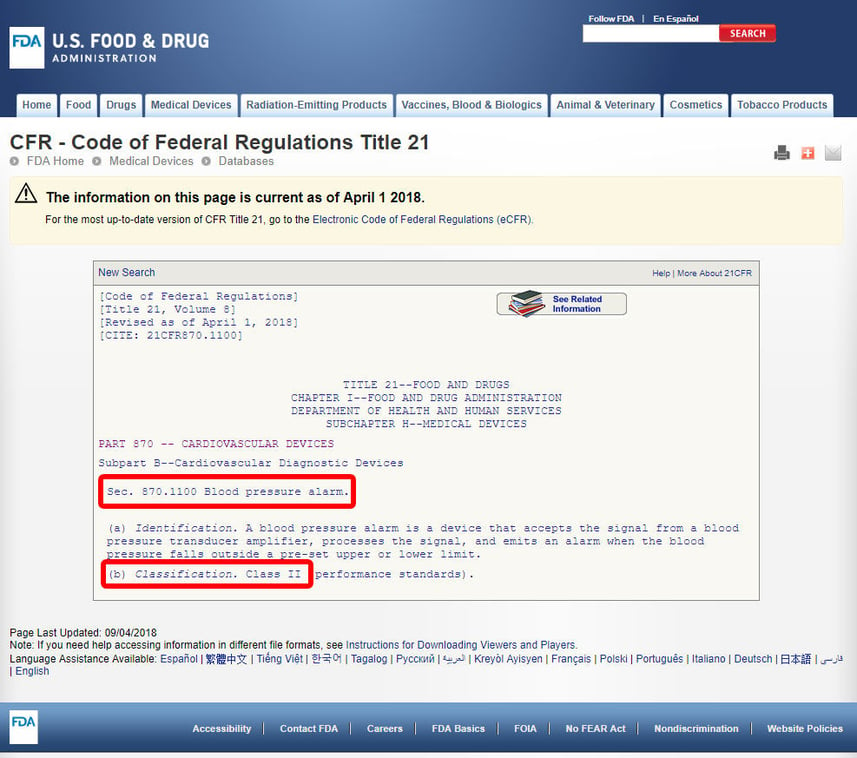This detailed screenshot captures a user's visit to the US Food and Drug Administration (FDA) website. In the top left corner, the FDA logo is prominently displayed, followed by the text "US Food and Drug" and "Administration" below it. The top section of the website is adorned with a blue banner that features a radiant gradient, transitioning from a lighter shade in the center to a darker hue on the edges. To the right of this banner is a search bar, accompanied by the text "Follow FDA" and "En Español" above it. The search button itself stands out in red.

Directly beneath the banner, a navigation menu provides quick access to various sections of the website, labeled Home, Food, Drugs, Medical Devices, Radiation-Emitting Products, Vaccines, Blood and Biologics, Animal and Veterinary, Cosmetics, and Tobacco Products. The specific page highlighted in the screenshot is titled "CFR - Code of Federal Regulations - Title 21." Below this title, there are breadcrumb links indicating the user's current path: FDA Home > Medical Devices > Databases.

A notable yellow caution banner warns that the information on the page is current as of April 1, 2018. Following this banner, a directed message appears, partially enclosed in a red-outlined rectangle, drawing attention to specific text. Additional information about the page's last update, notes, and language assistance options is provided below the message.

At the bottom of the screenshot, a secondary banner offers further links for navigating the website, ensuring users have access to a wide range of resources and information.